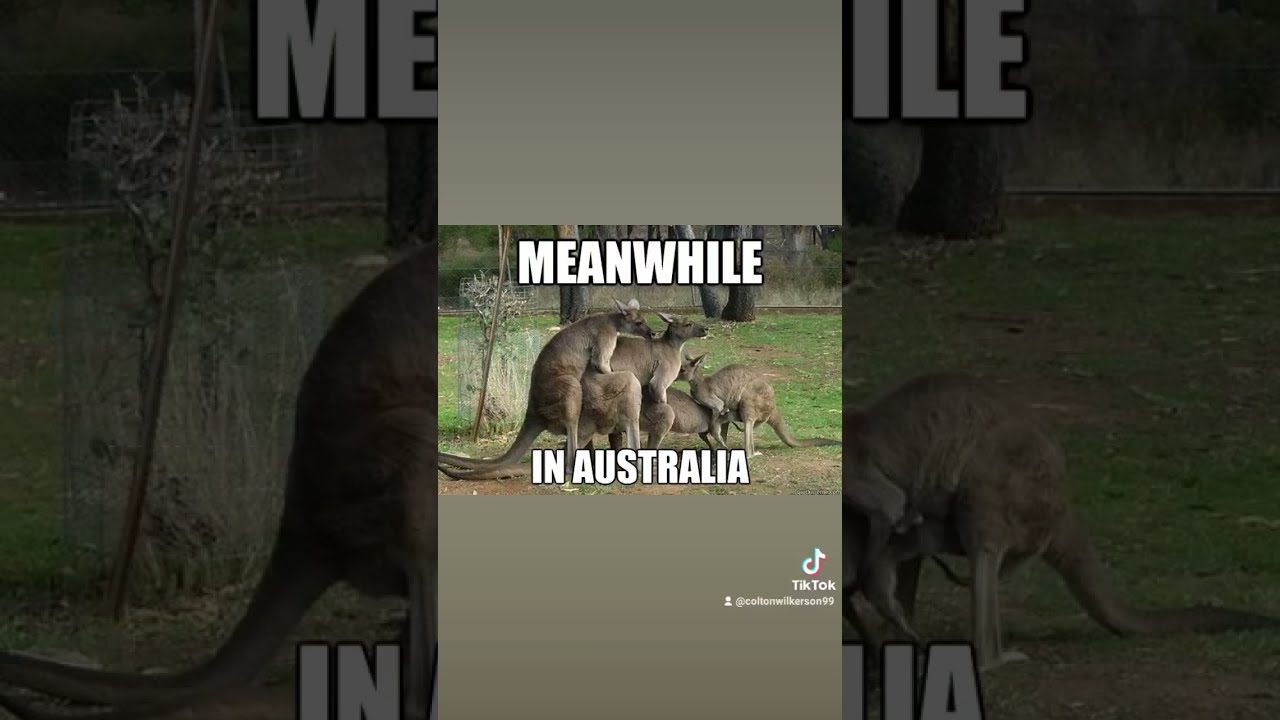The image is a composite of three sections: a bright center column flanked by two very tinted side columns. The central portion shows a quartet of kangaroos in an open grassy field with a few trees in the background. The text "MEANWHILE" is displayed at the top of the image in white uppercase letters, and "IN AUSTRALIA" is written beneath it in all capital letters. At the bottom right corner, the TikTok logo and the username of the poster are visible. 

In the center, there are four kangaroos lined up; the two on the left are larger and face to the right, while the two on the right are smaller and face the left. A flat gray surface is seen in front of them. The left tinted section zooms in on the tail of the leftmost kangaroo, while the right tinted section focuses on the smaller kangaroo on the right.